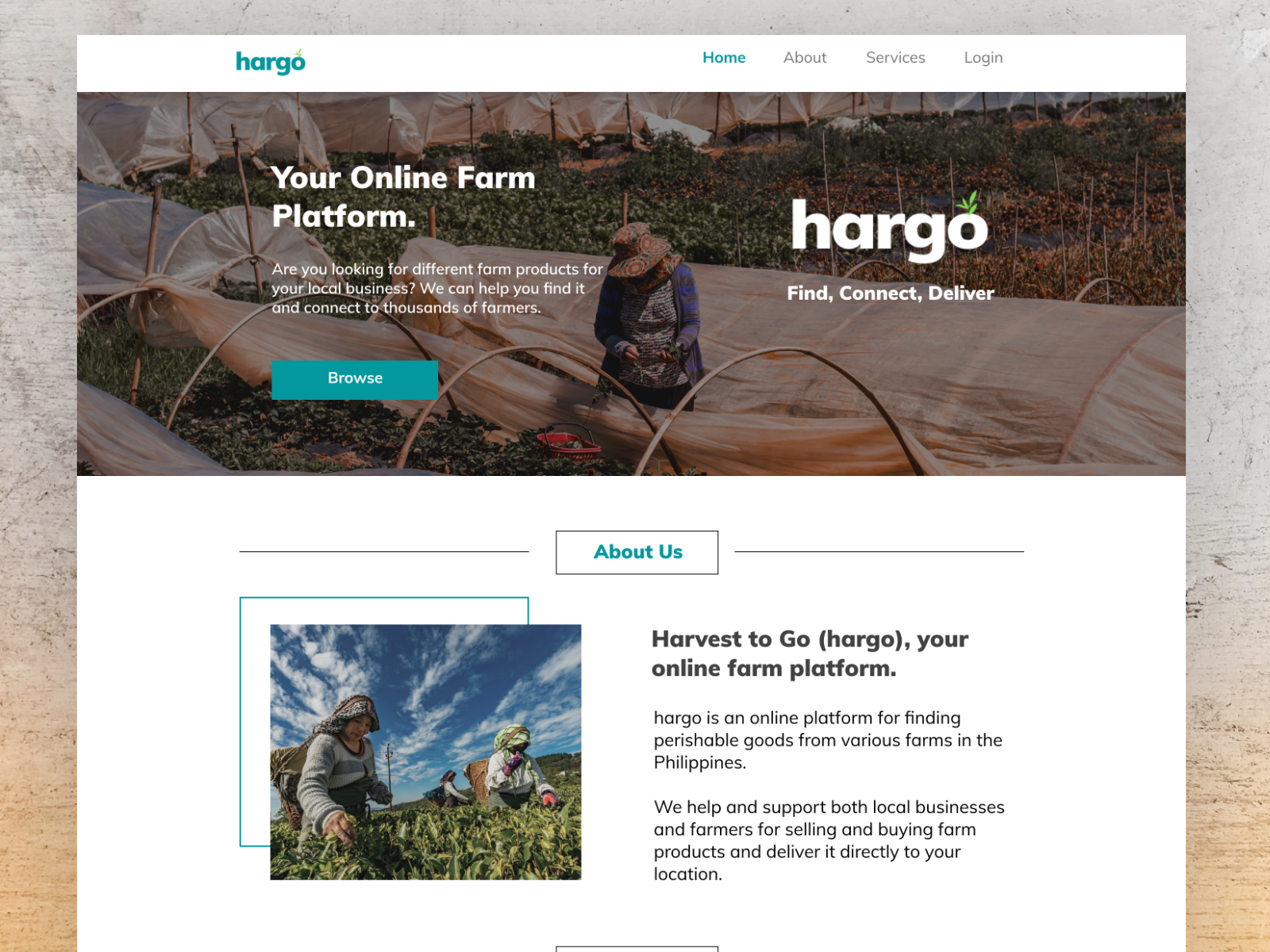This screenshot showcases the homepage of Hargo, an online farm platform. The background of the page features a photo, though it is obscured by other content elements. Dominating the page is a large white rectangle that nearly fills the entire screen. At the top of this rectangle, the word "Hargo" appears alongside navigation options: "Home," "About," "Services," and "Login," with "Home" highlighted in blue.

Below this header, a prominent image displays a person wearing a hat, tending to plants in an outdoor farm setting. The plants are partially covered with plastic, which has been peeled back in one area where the individual is working, possibly harvesting or caring for the crops.

Text beneath the image reads, "Your online farm platform. Are you looking for different farm products for your local business? We can help you find it and connect to thousands of farmers." A blue “Browse” button encourages users to explore further options.

To the right, the Hargo logo features a plant growing out of the “O” in "Hargo," accompanied by the words, "Find, collect, connect, deliver." 

The section below this, set against a white background, is titled "About Us." It includes a picture of people in a field harvesting vegetables. Next to the image, the text reads "Hargo. Harvest to go. Hargo, your online farm platform. Hargo is an online platform for finding perishable goods from various farms in the Philippines."